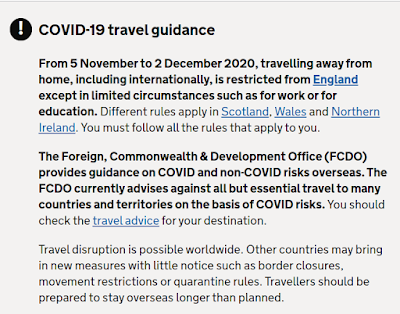The image displays a very light grey square with a black dot containing a white exclamation point in its upper left corner. To the right of this symbol, in bold black capital letters, it reads "COVID-19." Below that, it states in bold letters "Travel Guidance." Further down, in smaller type, it specifies: "From November 5th to the 2nd December 2020, traveling away from home, including internationally, is restricted from England except in limited circumstances such as for work or education." The words "restricted from England" are blue and underlined, and all text in this section is bolded.

The next line, in regular black type, says "Different rules apply in," followed by "Scotland," "Wales," and "Northern Ireland," all in blue, underlined, and separated by black text. It concludes with, "You must follow all the rules that apply to you."

In boldface type below, it reads, "The Foreign, Commonwealth & Development Office (FCDO) provides guidance on COVID and non-COVID risk overseas." The acronym "FCDO" and the words "COVID" and "non-COVID" are all in caps. It concludes by stating that the "FCDO currently advises against all but essential travel to many countries and territories on the basis of COVID risk."